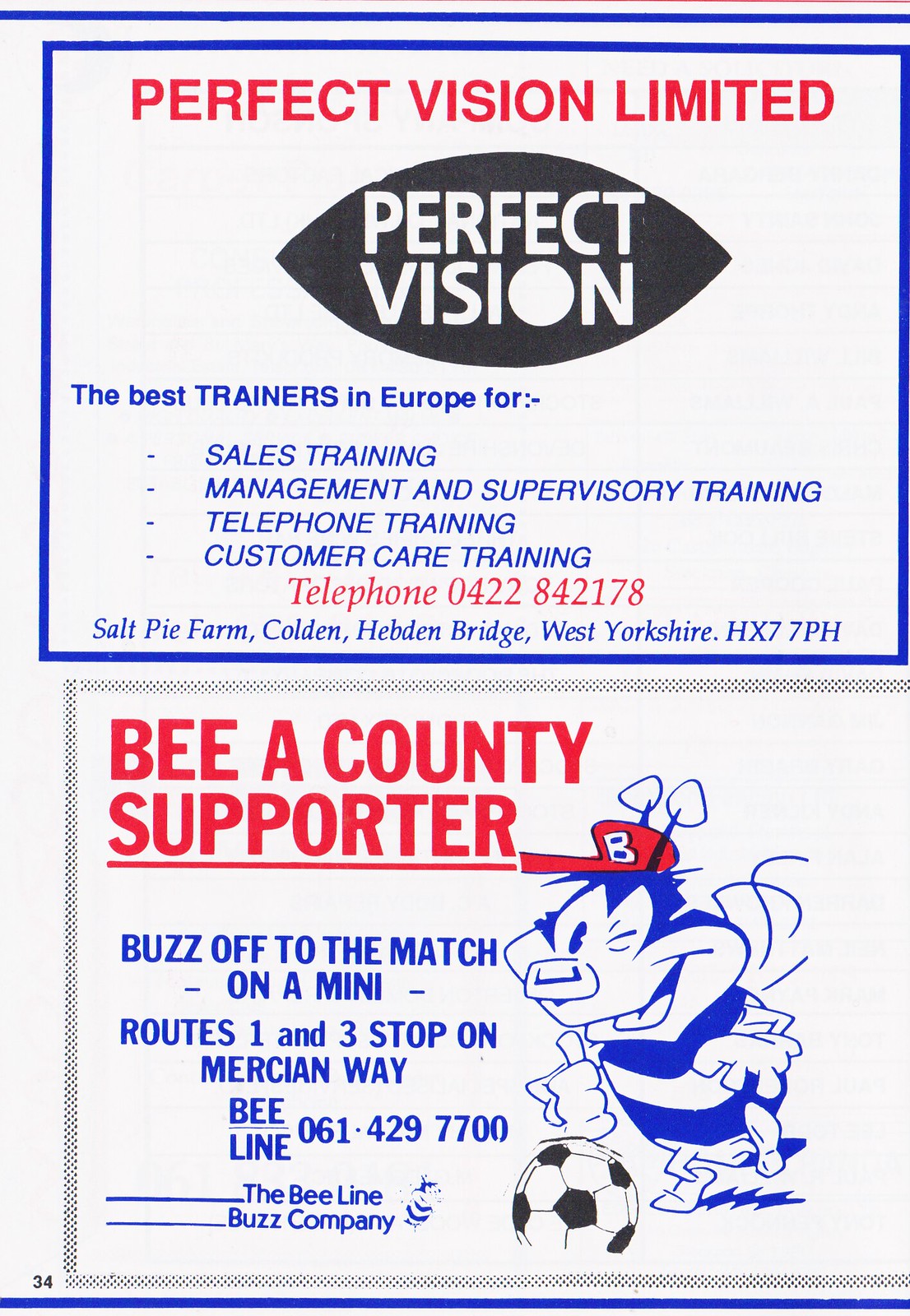This image exhibits two half-page advertisements, each with distinct branding and visual elements, likely from a catalog or magazine as indicated by the page number 34 at the bottom left. 

The top advertisement features a blue rectangular border and a white background. It prominently displays “Perfect Vision Limited” in red text at the top. At the center, a black eye logo contains the white text “Perfect Vision.” Beneath the logo, blue text highlights the company's expertise: "The Best Trainers in Europe for Sales Managed Training, Management and Supervisory Training, Telephone Training, Customer Care Training." A red contact number, 0422-842-178, is provided, along with the address in blue text: Salt Pie Farm, Colden, Hebden Bridge, West Yorkshire, HX7PH.

The bottom advertisement, also outlined in gray, has a white background and bold red text reading "Be A Conte Supporter," with “Be” creatively spelled as "B-E-E" to match the theme. An illustrated blue and white bee in a red hat, labeled "B," is depicted kicking a soccer ball. Blue text alongside instructs, "Buzz Off to the Match on a Mini, Routes 1 and 3, Stop on Mercy and Way," followed by contact information for the Bee Line Buzz Company at 061-429-7700.